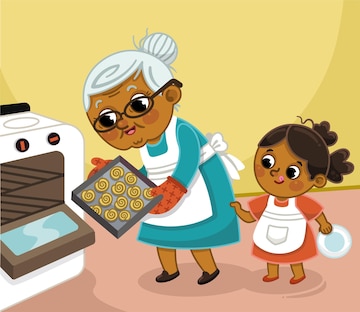The image is a colorful animated cartoon featuring a grandmother and her granddaughter baking in a kitchen. The scene is set against a plain yellow wall with a pink floor. To the left, there's a white oven with its door open. The brown-skinned grandmother stands next to the oven, slightly bent forward, as if she is placing or retrieving a tray of cinnamon rolls from the oven. She has white hair pulled back in a bun, wears dark glasses, a turquoise dress, a white apron, and red checkered oven mitts, paired with black shoes. 

The granddaughter, also brown-skinned, stands by her grandmother's side, smiling and holding the edge of her dress. She is wearing a pinkish coral dress with a white apron and red shoes, and her curly brown hair is styled in two ponytails. In her left hand, she holds a small white plate. Both characters have rounded faces and big eyes, contributing to the cutesy cartoon style of the image.